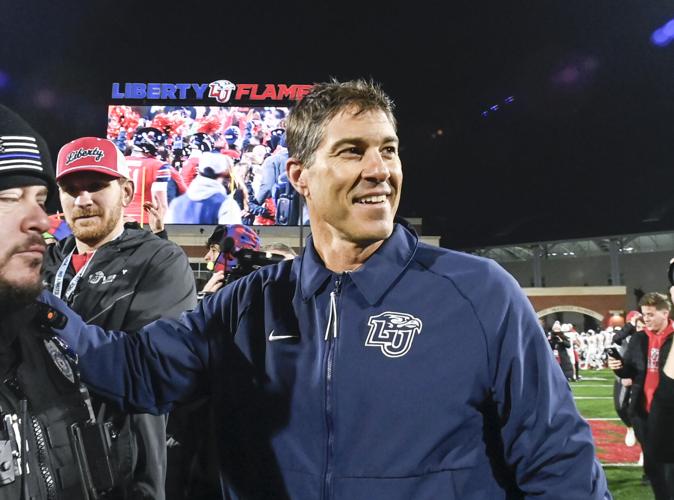The square photograph captures a vibrant nighttime football scene at a stadium. The dark sky above is dotted with a few blurred lights from the stands, adding to the nighttime ambiance. Dominating the upper background is a large jumbotron displaying "Liberty Flames" with "Liberty" in blue and "Flames" in red, along with a live image from the field. On the field, action from the game is visible, with players in white uniforms scattered around.

In the foreground, three men stand prominently. On the far left, partially in view, is a man with squinted eyes, possibly a security officer, wearing a black jacket embellished with a badge. Beside him stands another man wearing a red and white Liberty-themed baseball cap and a blue jacket. The main focus, however, is on the presumed coach at the forefront. The coach, with a broad smile and short brown hair, is clad in a dark blue collared jacket bearing a capital "LU" with an eagle insignia and a Nike logo. His hand rests casually on the shoulder of the man in the black jacket.

The detailed scene extends to the background where the vibrant green football field with distinct hash marks can be seen. Surrounding the field are other people, potentially cheerleaders and spectators, all contributing to the dynamic energy of the event. The stadium structure, including rafters and a walkway tunnel below, further frames this lively sports moment.